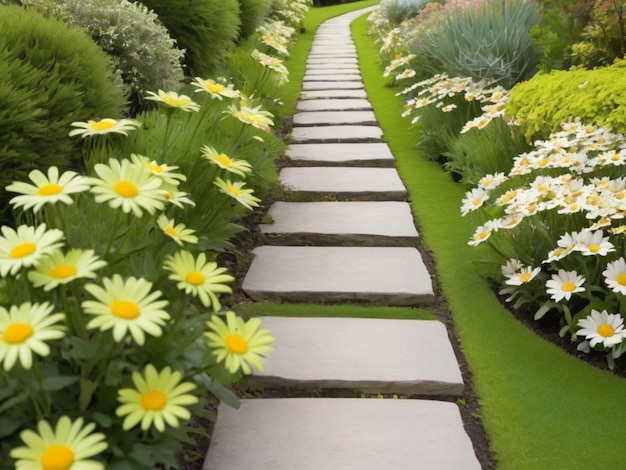The image depicts an almost surreal outdoor path that appears AI-generated due to its uncanny perfection. The pathway consists of a long row of thick, square cement steps interspersed with lines of dirt, grass, and greenery, extending from the bottom center of the scene and curving off to the right in the distance. The cement steps are unnaturally smooth and evenly laid out, giving them a suspiciously flawless appearance without crevices. 

To the left of the pathway, white petaled daisies with yellow centers line the edges, occasionally appearing with a greenish tint that adds to the image's surreal quality, alongside neatly trimmed bushes and various plants, possibly including wild herbs. On the right side, there is well-maintained grass, resembling a putting green in its perfect trim and texture. This side also features more perfectly white daisies, yellow-centered, framed by additional greenery and bushes, echoing the left side’s botanical setting. The entire scene could be from a high-end garden or botanical garden, enhanced with meticulous landscaping, yet the flawless elements suggest it might have been digitally rendered. The overall composition, with its pristine and manipulated look, combines elements of a picturesque garden path with an unnaturally perfect aesthetic.